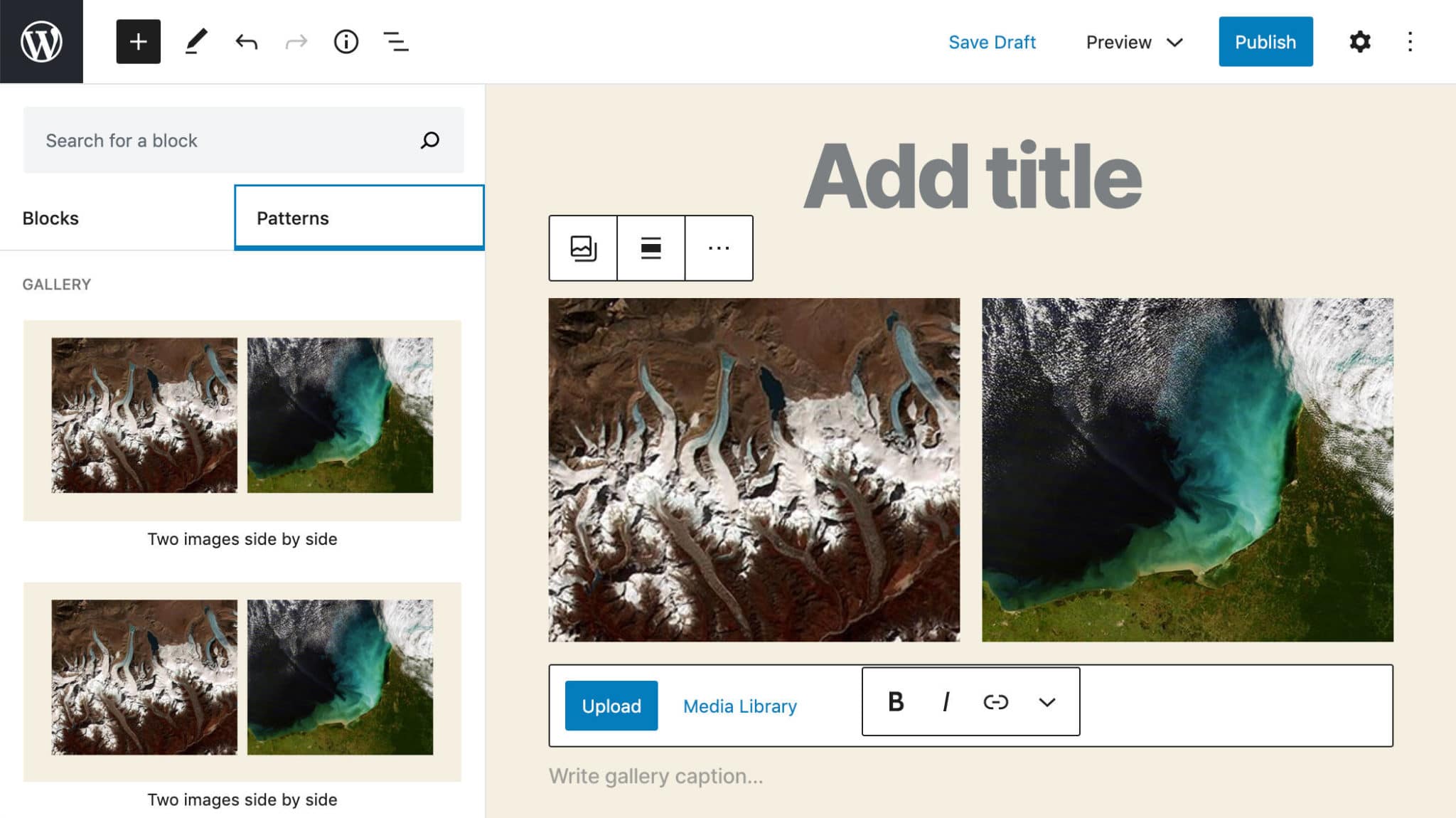The image depicts an interface of a website designed for publishing images. In the top left corner, the website is branded with a distinctive "W" symbol enclosed in a circle. On the top right, there are three prominent buttons: a blue "Publish" button, a "Preview" button in black letters, and a "Save Draft" option in blue letters.

The interface is clearly structured. In the left-hand sidebar, there are two categories: "Blocks" and "Patterns," with "Patterns" currently selected. Below this section, two images are displayed side-by-side; the first depicts a snow-capped mountain range, while the second shows a tranquil water area, possibly a lake or ocean.

The main working area of the site, situated to the right, offers a large space for editing and arranging content. At the top of this area, there is a placeholder for adding a title in large, bold blue letters. Below, there is a search bar for uploading images, accompanied by a "Media Library" button. This allows users to select images from their library, add titles, and write captions for their galleries before publishing.

Overall, the image illustrates a well-organized web interface that facilitates the comparison and management of images, with user-friendly options for adding titles and captions, and ultimately publishing the curated content.